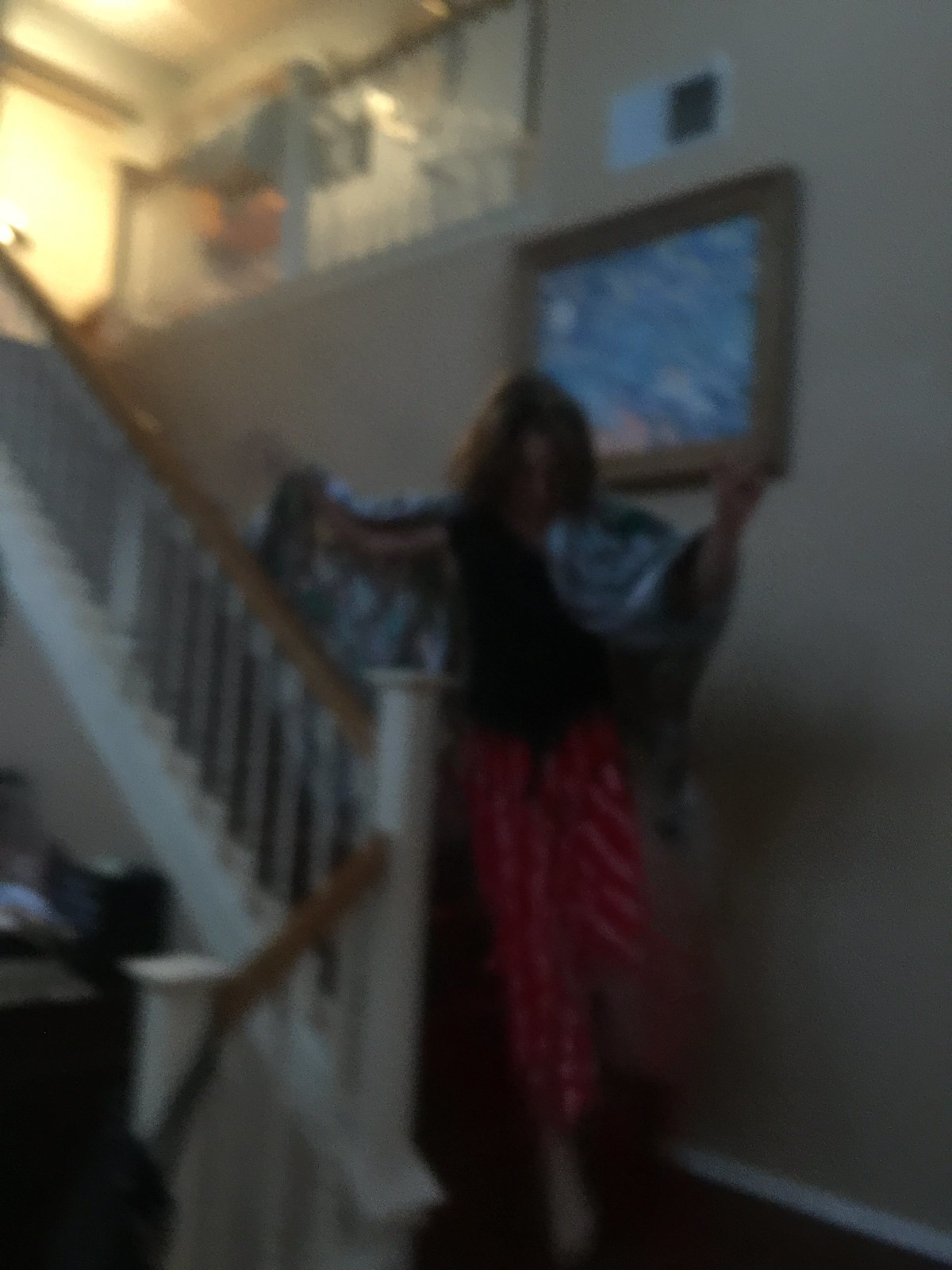In this blurry, low-resolution color photograph taken from the ground floor, a young person, possibly a woman or a child with long brown hair, is descending a stairway. The stairwell features white stairs with white spindles and a wooden handrail, alongside a beige wall adorned with a framed painting. The staircase is illuminated by light from the second floor, casting shadows on the bottom part. The person descending wears red pajama pants, potentially striped with pink or white, a black short-sleeved shirt, and has a blanket draped over their shoulders. They appear to be lifting their arms slightly, possibly adjusting the blanket.